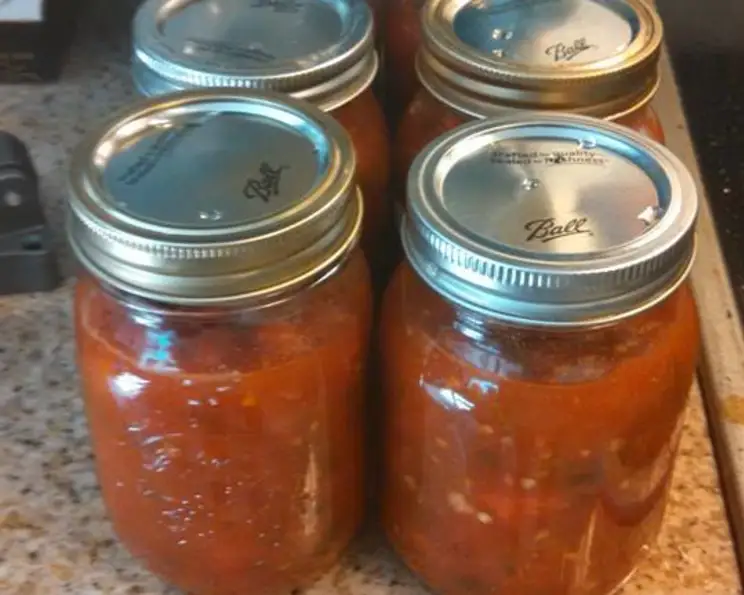In this photograph, there are four cylindrical, transparent mason jars neatly arranged in two rows on a cream-colored surface with black and white dots. Each jar has a classic round silver lid, which features the word "Ball" written in black script. The jars are filled with what appears to be a red sauce or semi-liquid substance, visible through the clear glass. There are a few yellow seeds suspended in the sauce, implying it might contain some tomato or pepper elements. The surface on which the jars are placed appears to be a beige or granite countertop, and there are other indistinct items to the left of the jars.